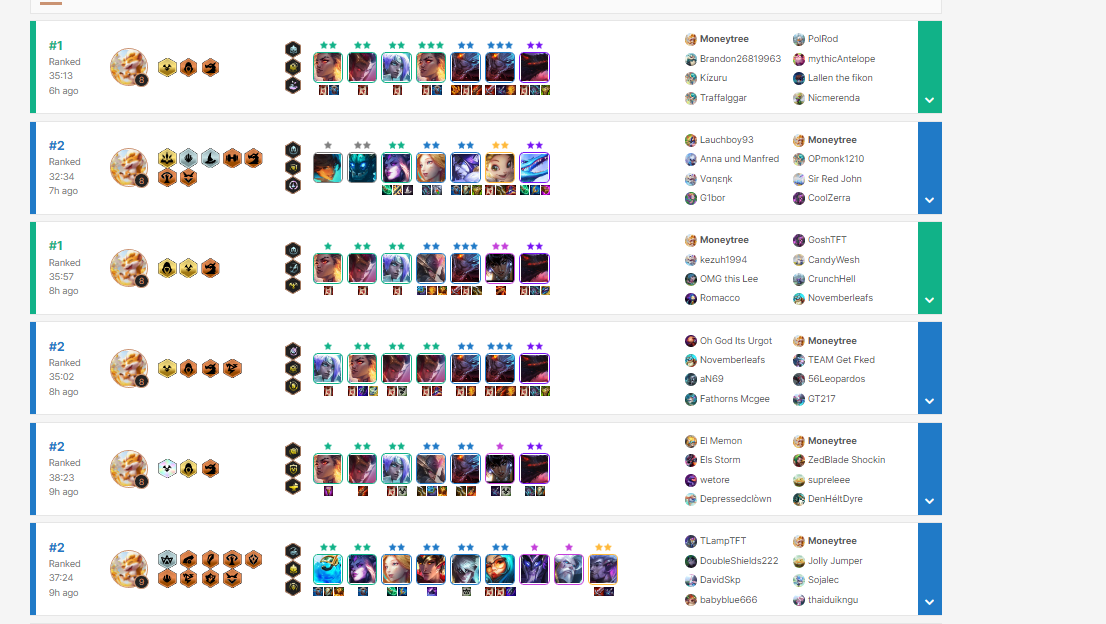This page, shrouded in mystery, appears to focus on the rankings of interactive games. It features six distinct rankings, with tiny, intricate text that makes it challenging to decipher. The page is adorned with numerous images of small creatures and devices, suggesting it might be a purchase page for web-based games. Notably, the highest-ranking slot showcases a collection of titles including "Brandon," "Kizuru," "Trafalgar," "Podrod," "Mythical Antelope," "Island," and "Nick Mirenda." The detailed imagery and array of names hint at an eclectic and engaging variety of game options available for enthusiasts.